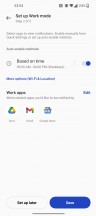This is a screenshot from a cell phone that is extremely blurry. When enlarged on a tablet screen, the image becomes even more distorted. In the upper left corner, it appears to display the time as 23:34, indicating 11:34 p.m. The battery icon in the upper right corner shows roughly 20% charge remaining. Next to the battery icon, there are signal indicators for cell phone reception and Wi-Fi, along with a few other indiscernible icons.

Immediately below, the text reads "Set up work," potentially followed by a date. There is some additional gray text underneath, including the word "based," though its context is unclear. A blue toggle switch, set to the "on" position, is visible below this line of text.

Beneath the blue toggle switch, additional blue text is present but illegible due to the blurriness. Further down, black text appears accompanied by what seems to be a blue "Edit" hyperlink to the right. Below this section, more gray text is visible, followed by a row of icons in the middle of the screen, including a recognizable Gmail icon, flanked by two other unidentified icons.